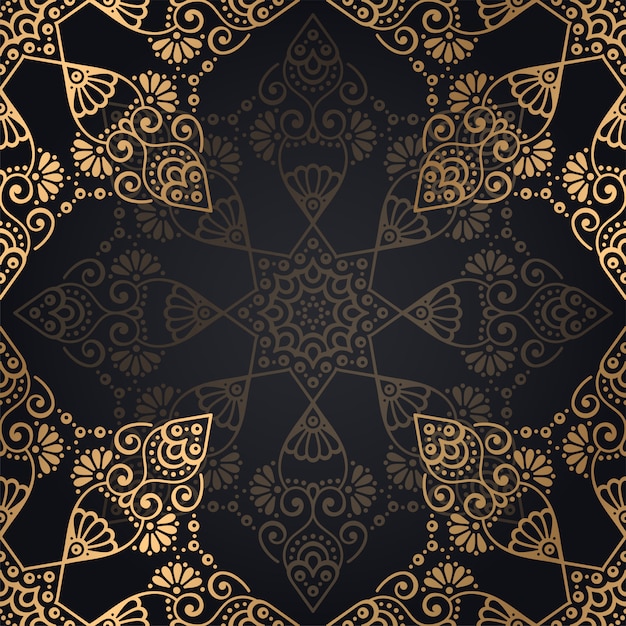This square image features a black background with varying shades that lighten towards the center, creating depth as the black gets progressively darker toward the edges. Overlaying this backdrop is an elaborate gold pattern that resembles paisley designs prominently placed in each corner. These corner designs include spirals, leaf shapes, circles, and arches, forming a decorative border that gives the impression of an abstract fish shape. The configuration of this pattern in the corners of the image leaves a central space that forms a cross-like shape with equal-length sides.

At the center of the image, a diamond-shaped pattern mimics the corner designs but is rendered in a more muted, lighter gold. This central design also contains elements suggesting curves, flowers, and dots, and when combined, these elements create an eight-pointed star, enhancing the intricate and symmetrical nature of the illustration. The play of light and shadow within the pattern produces a 3D effect, resembling a paper cut-out design. This intricate design might serve well as a background for graphic design work due to its detailed yet harmonious composition.